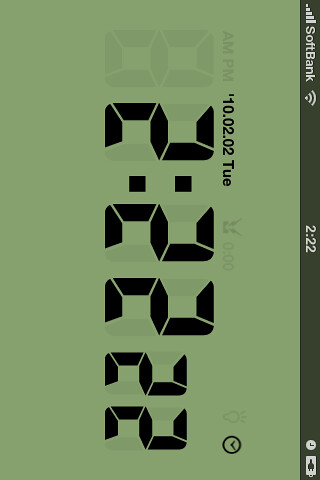The image is a screenshot of a smartphone's lock screen, displayed sideways with a green background. At the top, a dark gray, slightly transparent taskbar features a Wi-Fi indicator and the SoftBank logo on the left, with the battery indicator on the right. The digital time, displayed in black font, reads "10:02:02 TUE" above the central time display of "2:22:22" in black digital-style font, suggesting the use of a 24-hour format. The lock screen also includes a white circle and a battery icon with a black plug inside on the right side. The combination of digital elements and indicators confirms it is a smartphone clock app in military time.